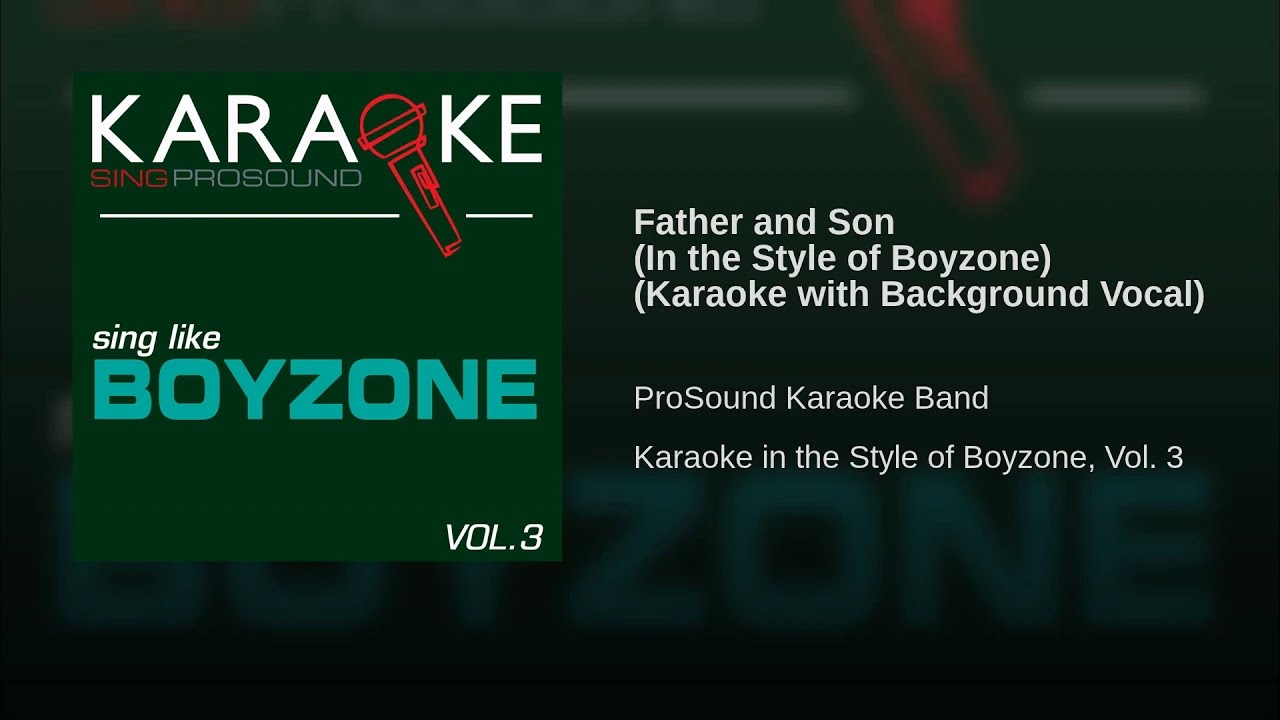The image is a computer-generated promotional flyer for a karaoke service, designed in a horizontal rectangular format with a business card-like shape. The central focus is a solid forest green square where the word "KARAOKE" appears in white capitalized letters, with the letter "O" cleverly replaced by a red microphone. Just below, it reads "Sing Pro Sound" and prominently features the phrase "Sing Like Boyzone Volume 3."

On the right side of the image, it displays additional information in white text, stating, "Father and Son in the style of Boyzone" along with the details "Karaoke with Background Vocal" and "Pro Sound Karaoke Band." The overall background is artistically blurred and zoomed in, replicating the album art, which adds a cohesive aesthetic to the design. This promotional image is reminiscent of YouTube music cover artwork or display graphics for music streaming services on TV or apps.